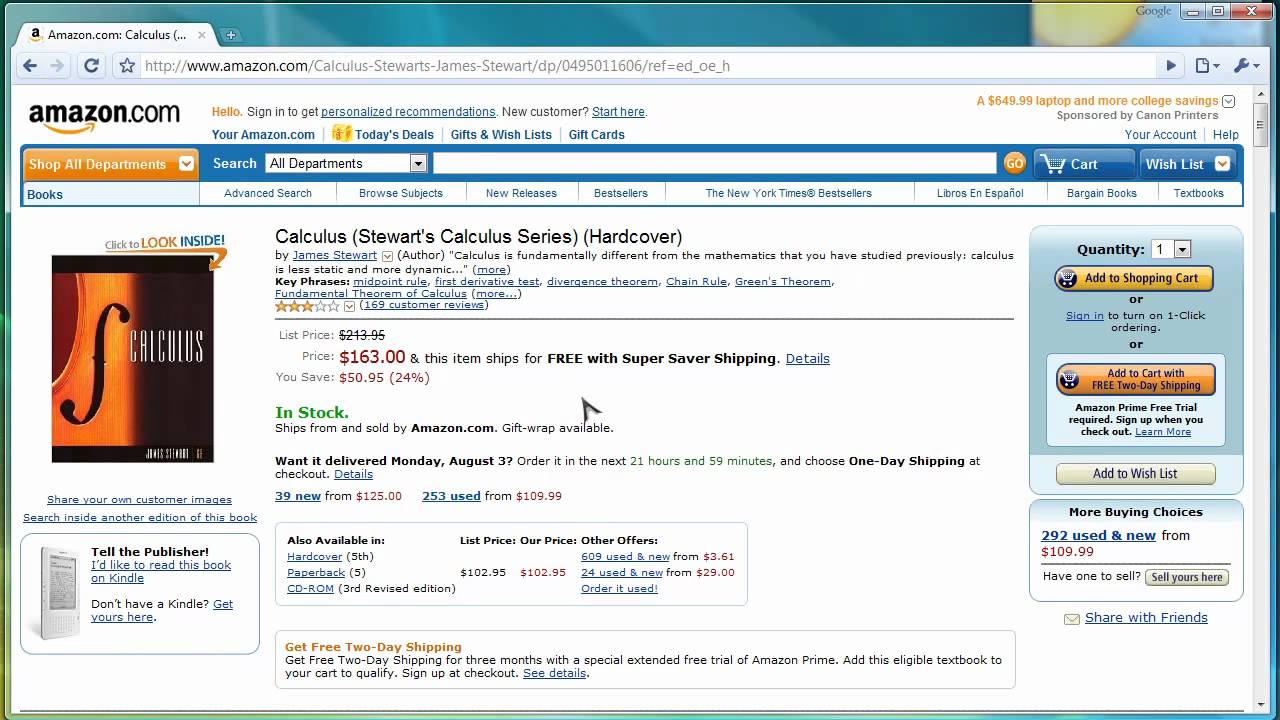The image depicts a computer screen showing a webpage from Amazon.com where a user is viewing a listing for a calculus textbook. The featured book is titled "Calculus" from Stuart's Calculus Series, authored by James Stuart. The description highlights that calculus is fundamentally different from previously studied mathematics, emphasizing its dynamic nature over static. Key phrases associated with the content of the book include the midpoint rule, first derivative test, divergence theorem, chain rule, Green's Theorem, and the fundamental theorem of calculus, among others.

The book has a three-star rating based on 169 customer reviews. It is priced at $163, with a noted discount of 24%, saving the buyer $50.95. The listing ensures potential buyers that the item is in stock and available for free shipping with the Super Saver option. The product ships from and is sold by Amazon.com, with gift wrapping available. At the top of the page, there is an option to "Click to Look Inside," allowing a preview of the book's content. Various interactive elements are visible on the screen, including buttons to "Add to Shopping Cart," "Add to Cart with Free Two-Day Shipping," and several other clickable areas.